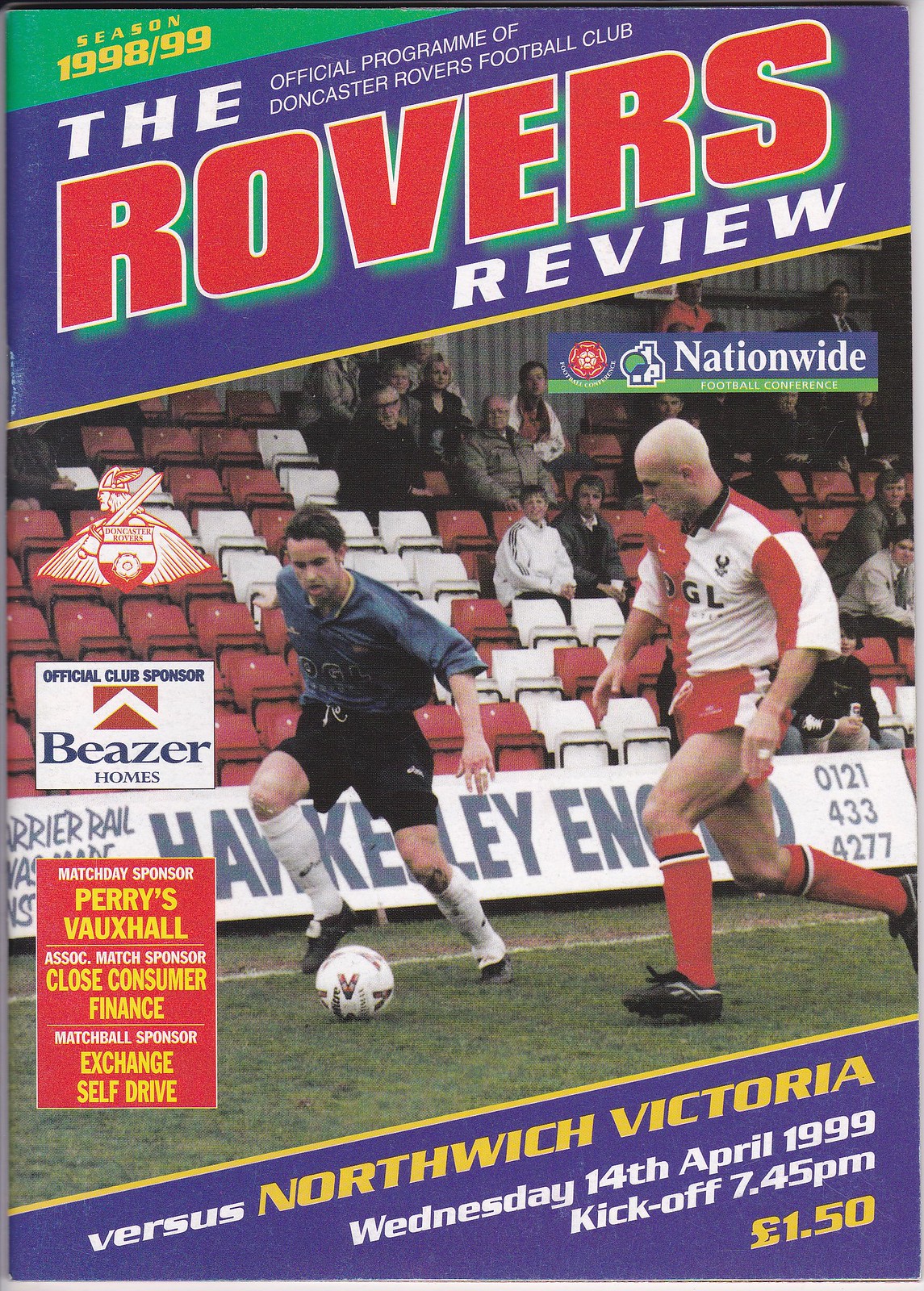The program cover for a soccer match features a green elongated triangle in the upper left corner with yellow text reading "Season 1998/99." Below, on a purple background, it states "The Official Program of Doncaster Rovers Football Club," with the prominent, bold red title "Rovers" and the word "Review" in white below it. A yellow line separates this section from the next. The central portion showcases an image of two players engaged in a soccer game in front of a crowd. The player on the right, donning a white and red jersey, red shorts with white accents, red socks, and black shoes, faces a shorter player on the left who wears a blue shirt, black shorts, and white socks with a soccer ball at his feet. Also, a team decal featuring a Viking head with a sword over the shoulder is visible to the left of the blue-shirted player. Below this, on a purple background, it indicates the match details: “Versus Northwich Victoria, Wednesday 14 April 1999, Kickoff 7:45 PM, £1.50.” Additional sponsors and logos are shown at the bottom: a white square for "Official Club Sponsor Beezer Homes" and an orange rectangle listing other sponsors: "Match Day Sponsor Perry's, Vauxhall Association, Match Sponsor Close Consumer Finance, Match Ball Sponsor Exchange Self Drive."